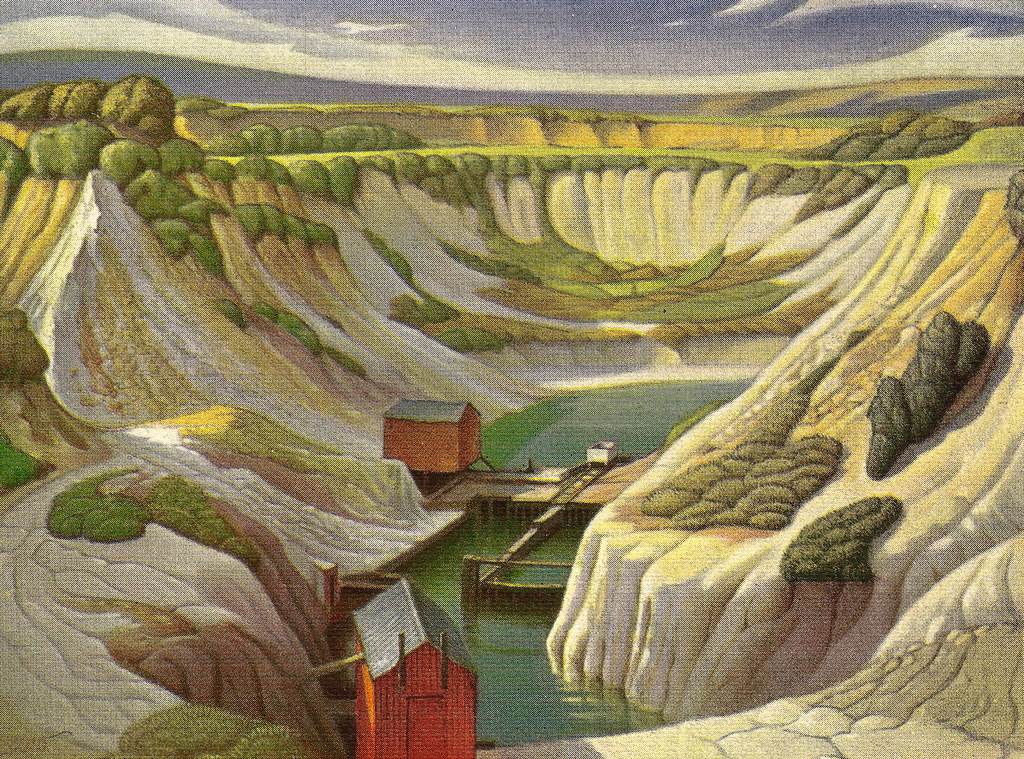This detailed illustration, reminiscent of artwork found in older books, depicts a deep, dugout quarry landscape with intricate textures that imply it was rendered on a rough canvas. Central to the scene is a green waterway flanked by white, tan, and light yellow rock formations, transitioning to areas of vegetation and plant life at the higher edges. Prominently, there are two identical barn-like red shacks with gray roofs; one is situated on a flat wooden platform on the left side of the waterway, and the other occupies the foreground's center-bottom. The scene is framed by surroundings of grassy patches on rocky hillsides and distant sand-toned hills and mountains. The sky overhead is portrayed in shades of gray with long streaks of white clouds, adding depth to this detailed illustration.